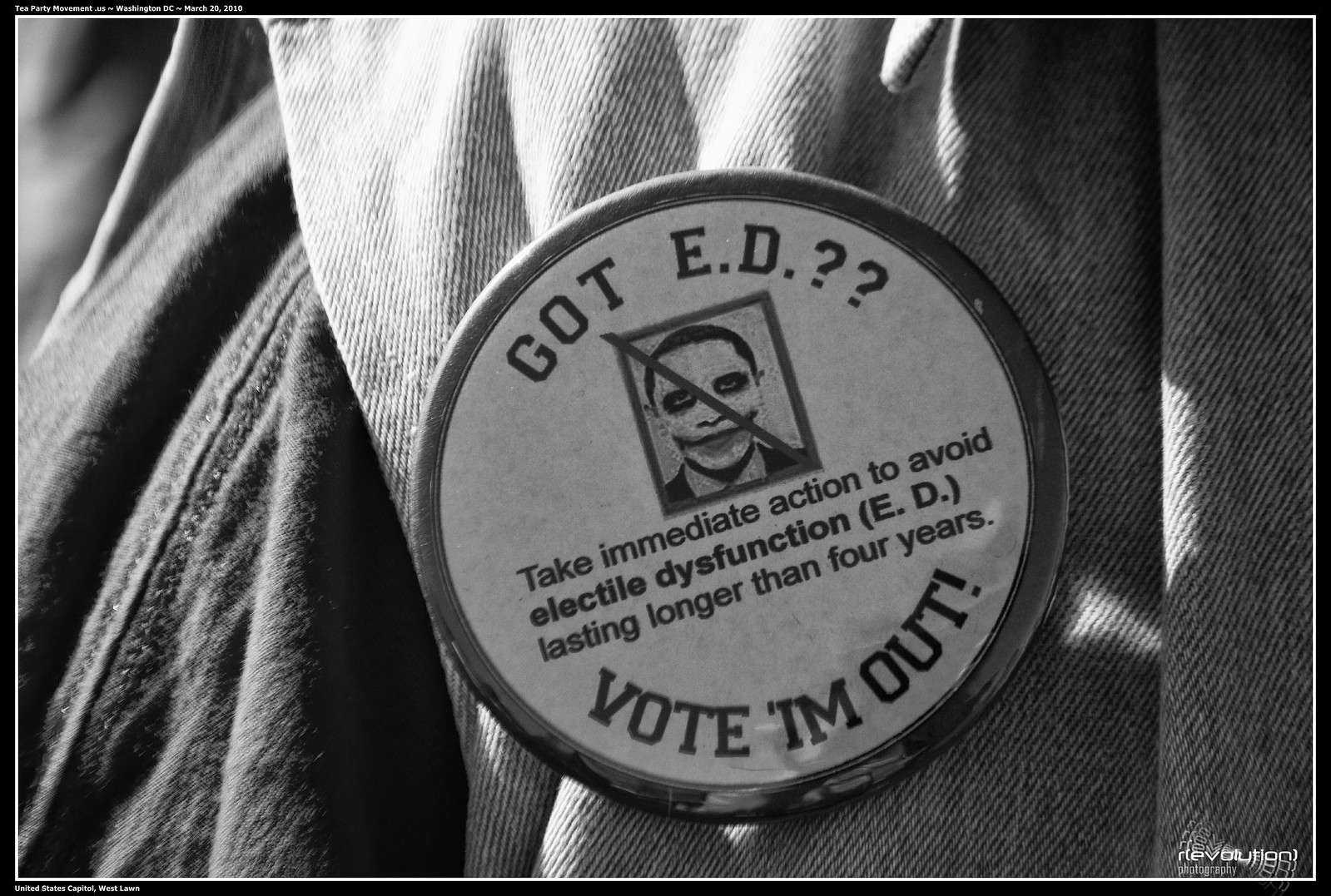The image showcases a solid black border with an interior white border framing the entire scene. Dominating the center is a piece of denim fabric, likely a coat, on which a prominent pin is attached. The pin features a satirical design with a picture of a man in Joker makeup, crossed out. Text on the pin reads, "Got ED? Take immediate action to avoid erectile dysfunction (ED) lasting longer than four years. Vote I'm out!" The words "Got ED?" are curved along the top of the circle, while "Vote I'm out!" is curved along the bottom. The entire image, including the denim and the pin, is rendered in black, white, and various shades of gray, suggesting a monochromatic theme likely intended for social media sharing.